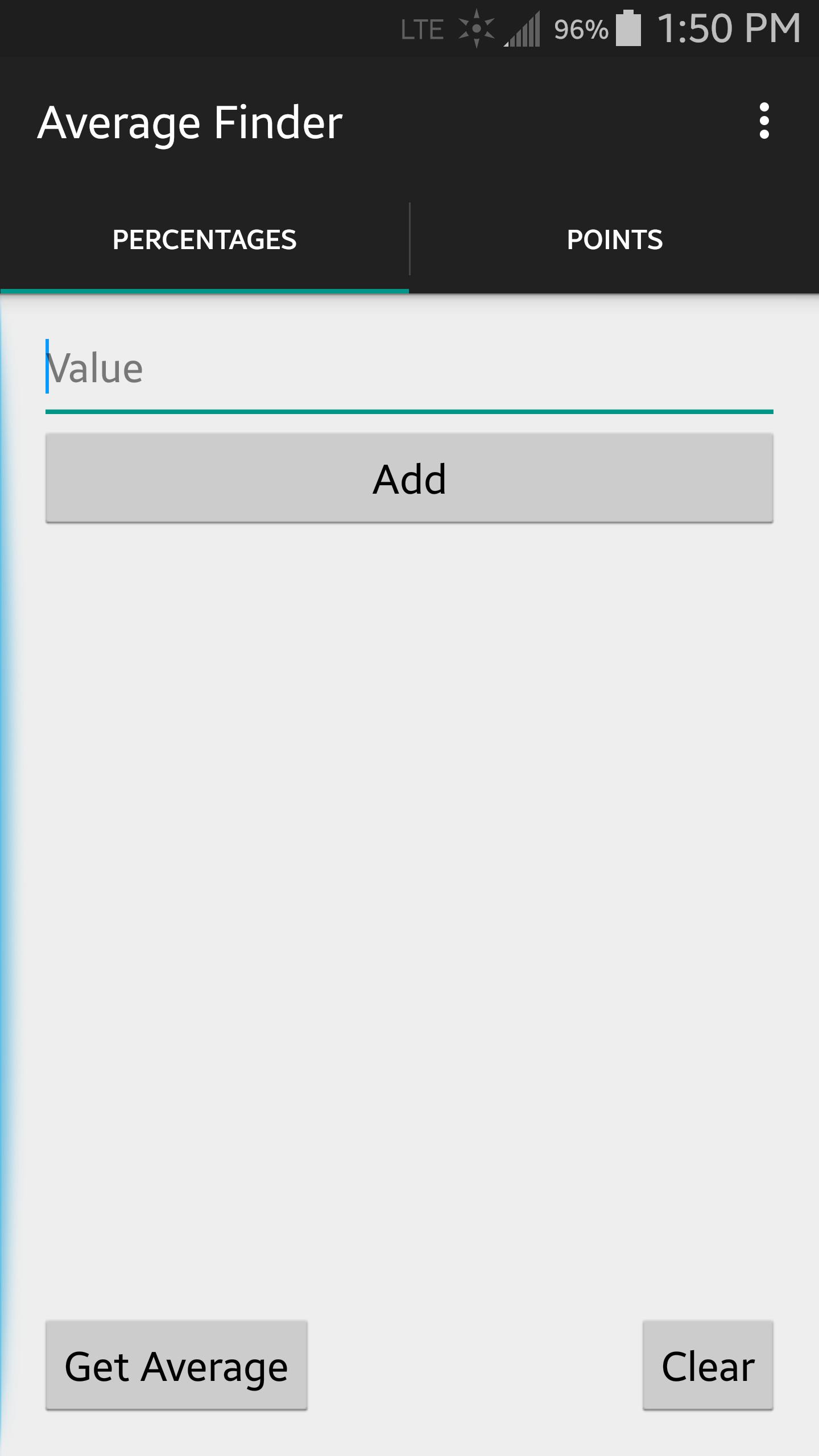The image showcases a smartphone app displayed in portrait orientation. At the top, there is a black bar occupying approximately one-fifth of the screen, featuring white text. Positioned towards the left-center of this bar, the text reads "AVERAGE FINDER." Below this title, there are two buttons: one labeled "PERCENTAGES" on the left and the other labeled "POINTS" on the right, both in white lettering.

Above the black bar, the phone's status indicators are visible, including the current time, a battery icon, and signal strength bars.

Below the black bar, the app's interface has a light gray background displaying the word "VALUE" aligned to the left. A teal line stretches horizontally across below this text. Underneath the line, there is a slightly darker gray button spanning almost the entire width of the screen, with the word "ADD" displayed in black text.

At the bottom of the screen, two additional buttons are present: one on the left labeled "GET AVERAGE" and another on the right labeled "CLEAR."